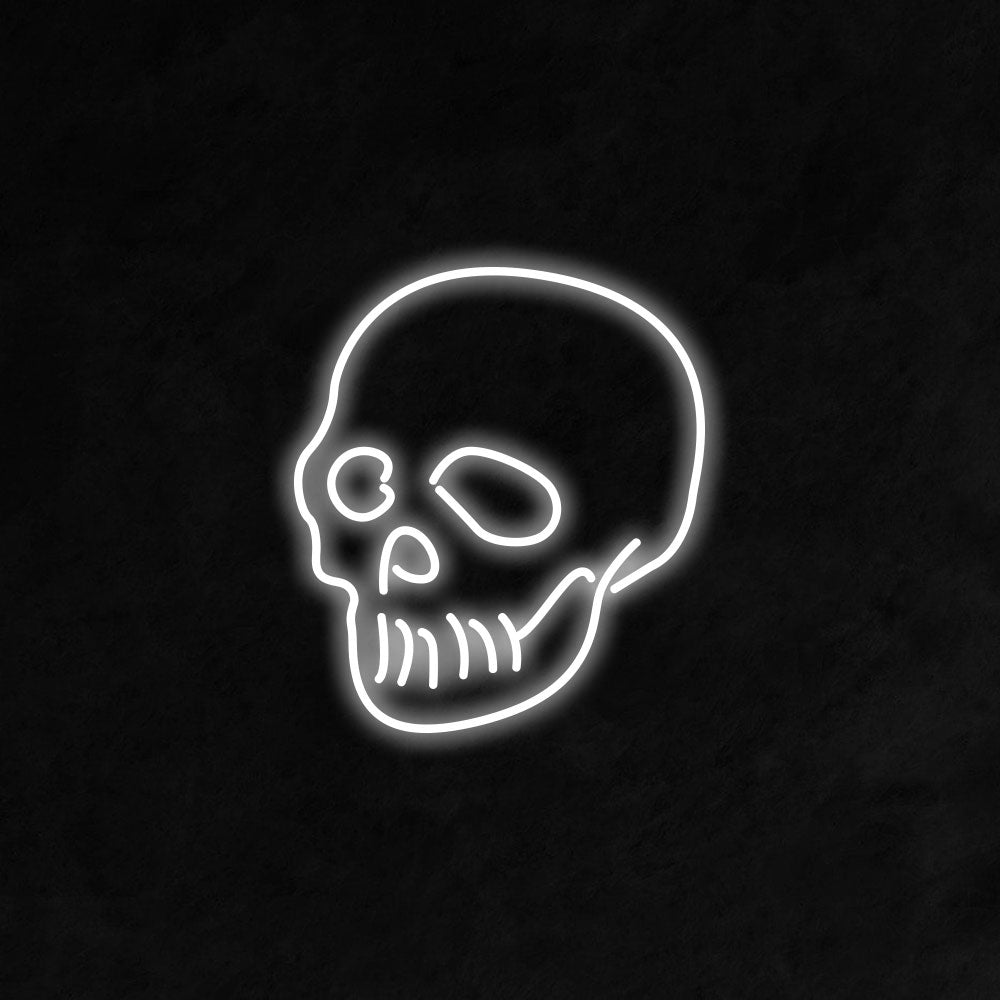Against a textured, charcoal-black background with grayish accents, a striking neon-like line drawing commands attention. This artwork features a human skull, rendered entirely in glowing white lines that give the impression of neon lights. The skull, placed precisely in the center of the piece, faces slightly to the left, showing its circular eye sockets, a squiggly nose, and lines for a closed mouth that suggest it is sewn shut. The minimalist composition—devoid of text or additional elements—emphasizes the skull's ethereal, luminescent presence against the velvety dark backdrop.